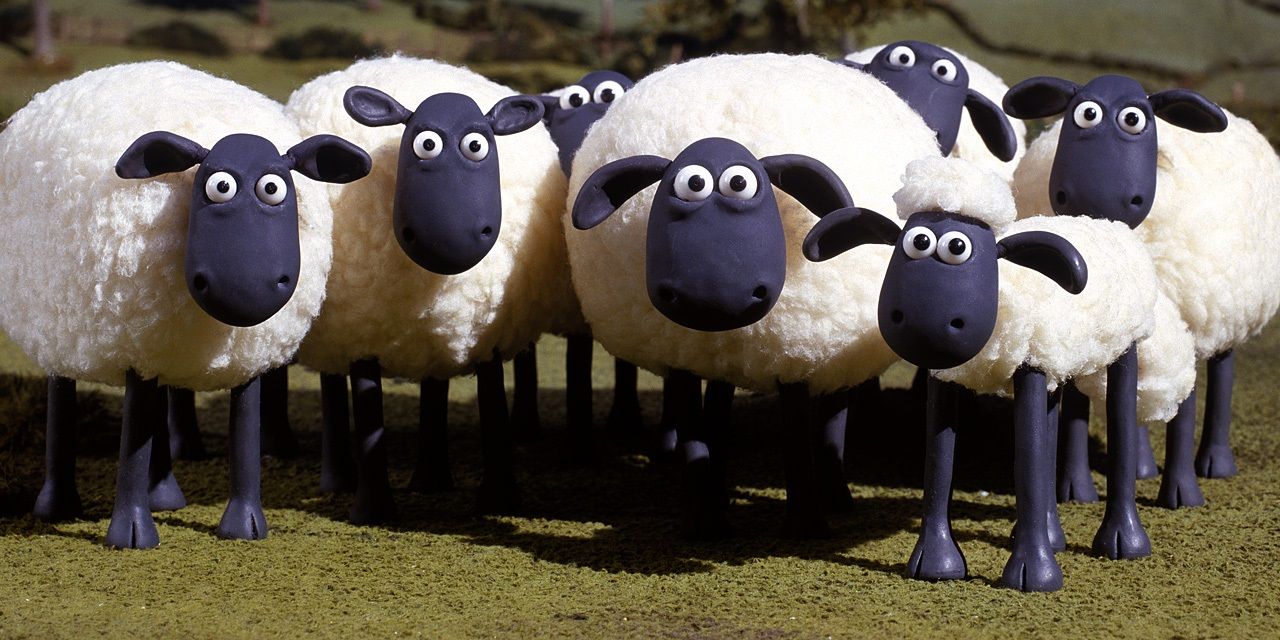The image depicts a humorous scene from the animated series Wallace and Gromit, featuring half a dozen sheep with distinctly white, fluffy bodies and black legs and heads. Their large, expressive eyes are white with black pupils, and they all appear to be staring directly at the camera. The sheep are arranged on a short-cut field of vibrant green grass. The central sheep is the most prominent, being very large and round, flanked by a slightly smaller sheep to its left and a smaller baby sheep to its right. The remaining sheep, although partially obscured, are situated in the background, peeking through the blurred backdrop of green bushes and hills, adding a playful depth to the scene. The playful depiction of the sheep and the richly detailed natural setting contribute to the overall whimsically animated charm.